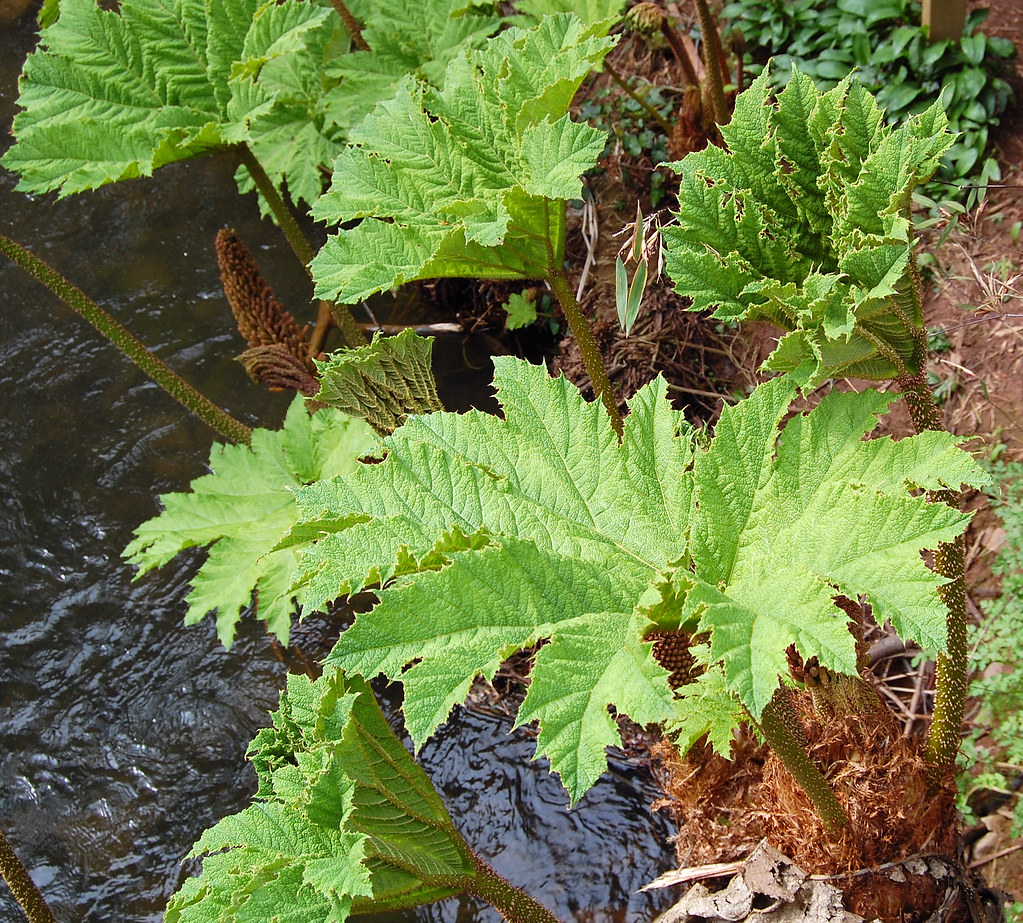The image captures a detailed and intimate view of a natural setting near a water body, likely a stream or creek, positioned to the left. The water appears slightly choppy but without pronounced waves. In the foreground, various leafy green plants dominate the scene, with some brown and darker leaves interspersed among them. The plants, with their prickly, cactus-like edges and stems, rise from a mixture of dirt and orange-ish, dead grasses. These elements are primarily centered in the image, creating a rich tapestry of green, brown, and yellow tones with hints of tan and red. The image appears slightly rotated counterclockwise, lending an artistic angle to the outdoor setting, which seems to be captured in the middle of the day.